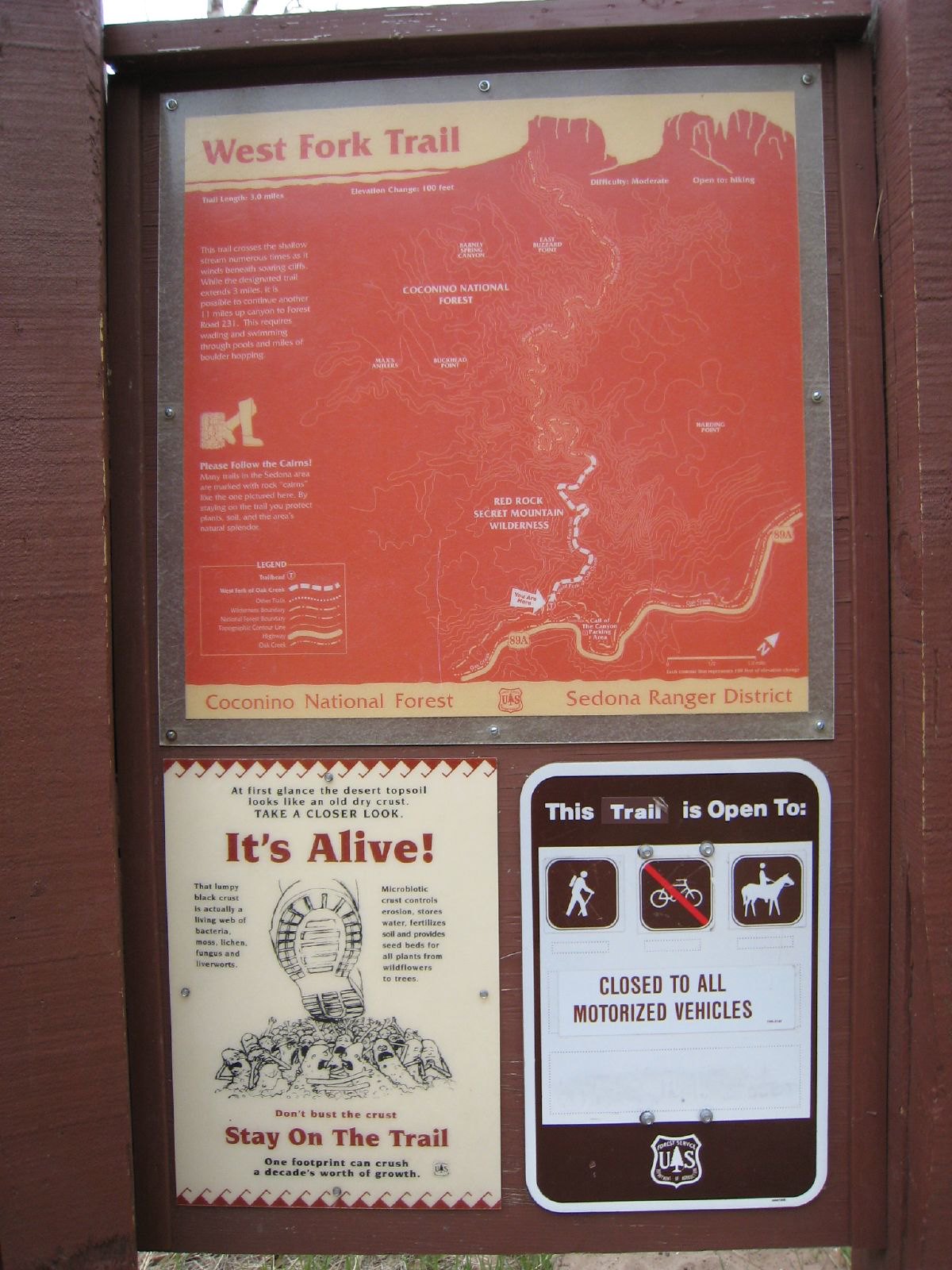The image is a daylight photograph of a detailed, vertically aligned rectangular sign set in a large brown painted wooden display within a nature park, specifically the Coconino National Forest, Sedona Ranger District. The top portion features a durable plastic-covered map titled "West Fork Trail," displaying yellow and red hues with red lettering and white text, too small to read. The map illustrates various trails, with some curving toward the mountains. Below the map is a white vertical sign with bold red text stating "It's Alive" at the top and "Stay on the Trail" at the bottom. In the middle of this white sign, there's a black and white illustration of a foot stepping on small creatures, along with text emphasizing the importance of staying on the trail to protect fragile desert life. In the lower right corner, another sign warns "Closed to All Motorized Vehicles" in red letters. At the top of this sign, it reads, "This trail is open to," followed by three squares depicting a walker, a bike with a red slash through it, and a person on a horse, indicating that the trail is accessible to walkers and horseback riders but not to cyclists. The wooden display is supported by posts on either side and contains informative signs to guide park visitors responsibly.